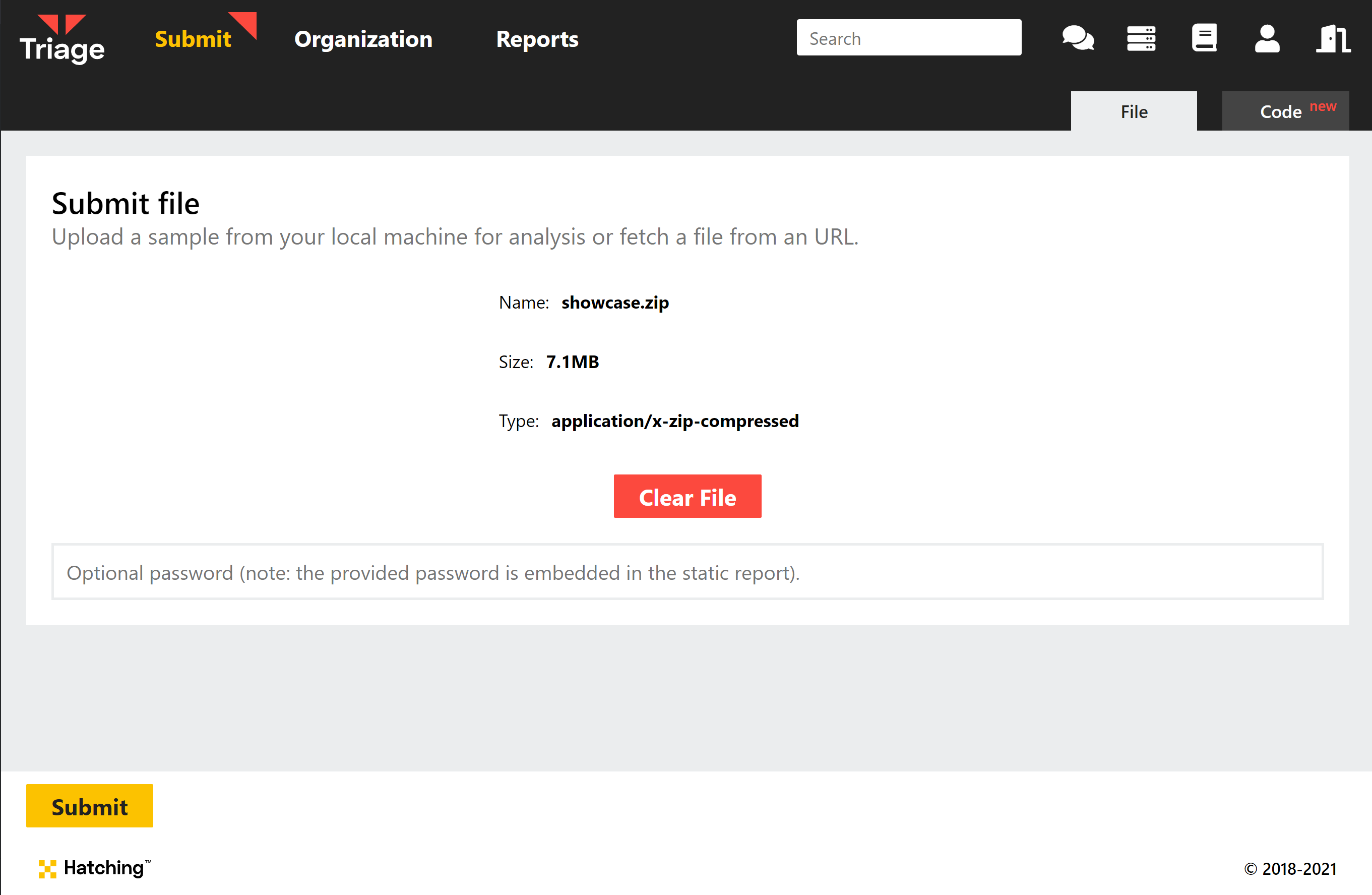Here is a cleaned-up and detailed descriptive caption for the image of the Tri-Edge website:

---

The image showcases the Tri-Edge website interface. In the top left corner, there are two red triangles adjacent to each other. Below these triangles, the Tri-Edge logo is prominently displayed in white letters, spelling out "TRIGE." To the right of the logo, three navigational tabs are visible: 'Submit,' marked with a small red triangle in its upper right corner; 'Organization;' and 'Reports.' Further right, a search box is situated next to a sequence of icons including a chat icon, a tab management button, a book icon, a user profile icon, and a door symbol which likely represents the log out button.

Below the navigation bar, on the right side, are the 'File' and 'Code' sections. Dominating the central part of the interface is a white box labeled 'Submit File.' The instructions in this section prompt the user to upload a sample file from their local machine for analysis or fetch a file from a given URL. A file named 'Showcase.zip' is shown, with its details listed as 7.1 MB in size and classified under the type 'Application-X-Zip-Compressed.' Adjacent to this information is a red button labeled 'Clear' designed to remove the file. Below, there's an optional field to input a password and, in the bottom left corner, a blue 'Submit' button to finalize the upload process.

---